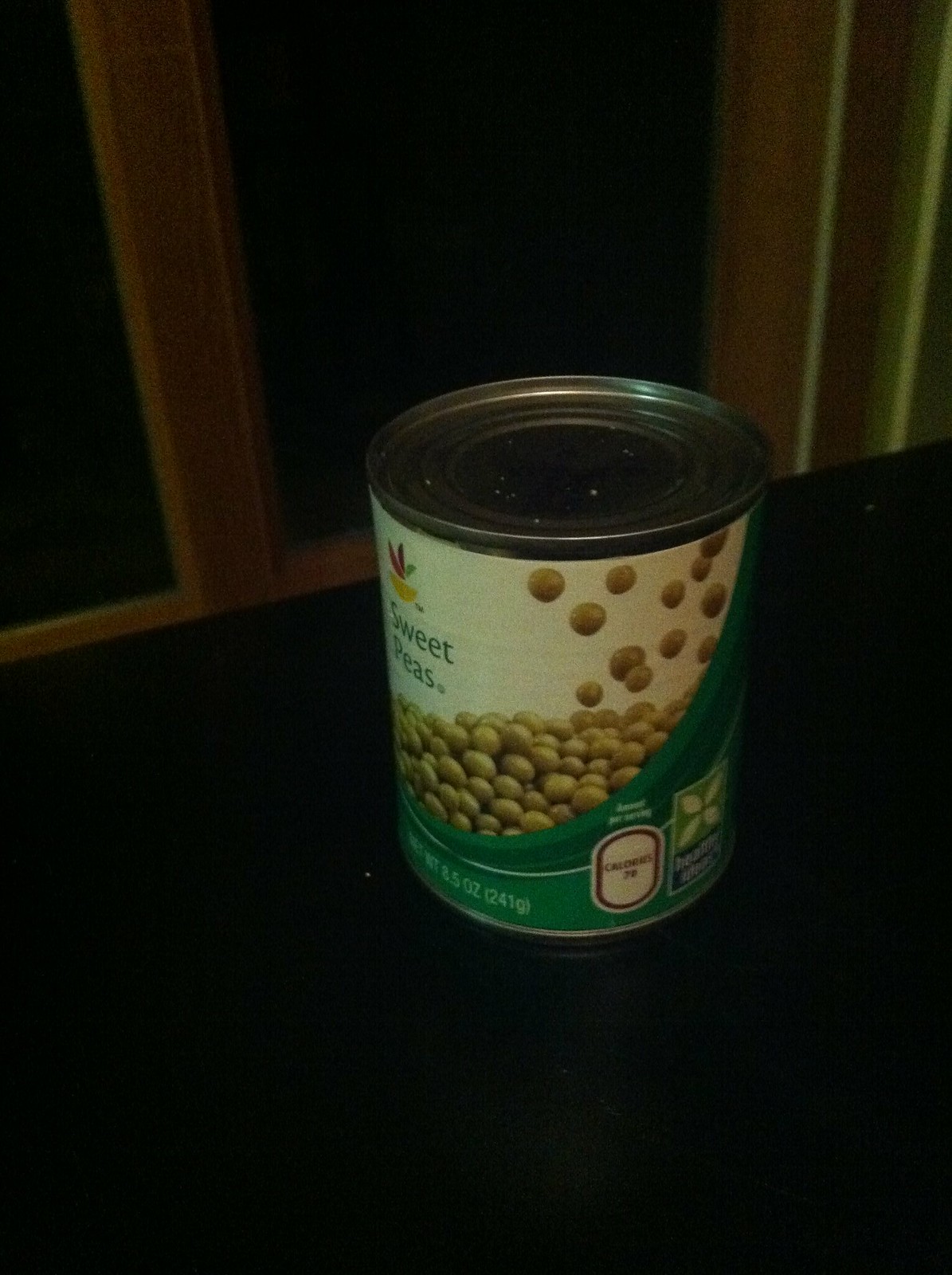This image captures a small, 8.5-ounce (241g) tin can of Stop-and-Shop Sweet Peas, prominently displayed on a dark wooden table with a wood-framed window in the background. The can's label features a vibrant, detailed design: at the top left, there is a yellow bowl with a reddish-orange leaf, a dark purple middle, and a lime green right section, signifying the Stop-and-Shop logo. Below this, in a traditional blue font, it reads "Sweet Peas" with both the "S" and "P" capitalized. The main body of the label shows a substantial pile of light green peas with additional peas cascading down into the pile, set against a white background with a stylized green swoop from the bottom left to the top right. The net weight is subtly displayed at the bottom in small, white font against a green backdrop. Additionally, the can is noted to be dusty on top, adding a touch of realism and detail to the scene.